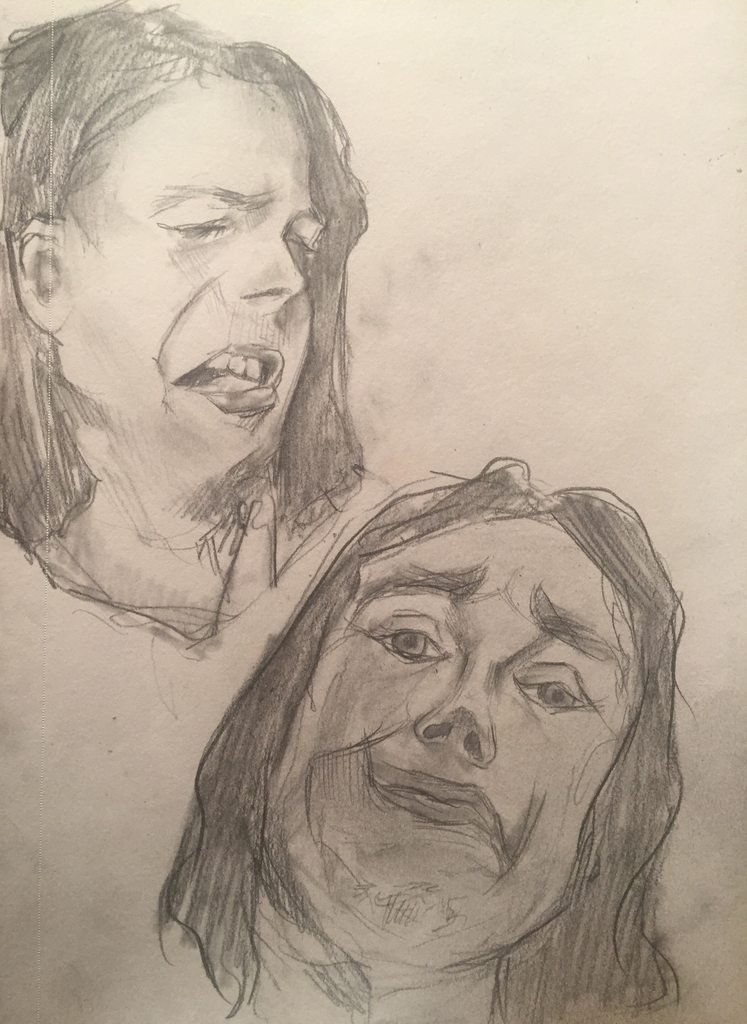A detailed pencil sketch on a white sheet of paper portrays the same female subject in two distinct expressions. The upper drawing presents a side profile of the woman's face from the left, with her eyes closed and appearing slightly squinted. She possesses straight, shoulder-length hair and displays an open mouth, suggesting an upset or distressed emotion. In contrast, the lower drawing offers a frontal view of the same woman. Here, her eyes are open, and her mouth is closed, with her eyebrows slightly raised in the middle, hinting at a sense of anguish or grief. Her hair is parted in the middle, cascading straight down on both sides. The artwork powerfully conveys a narrative of emotional suffering through detailed facial expressions.